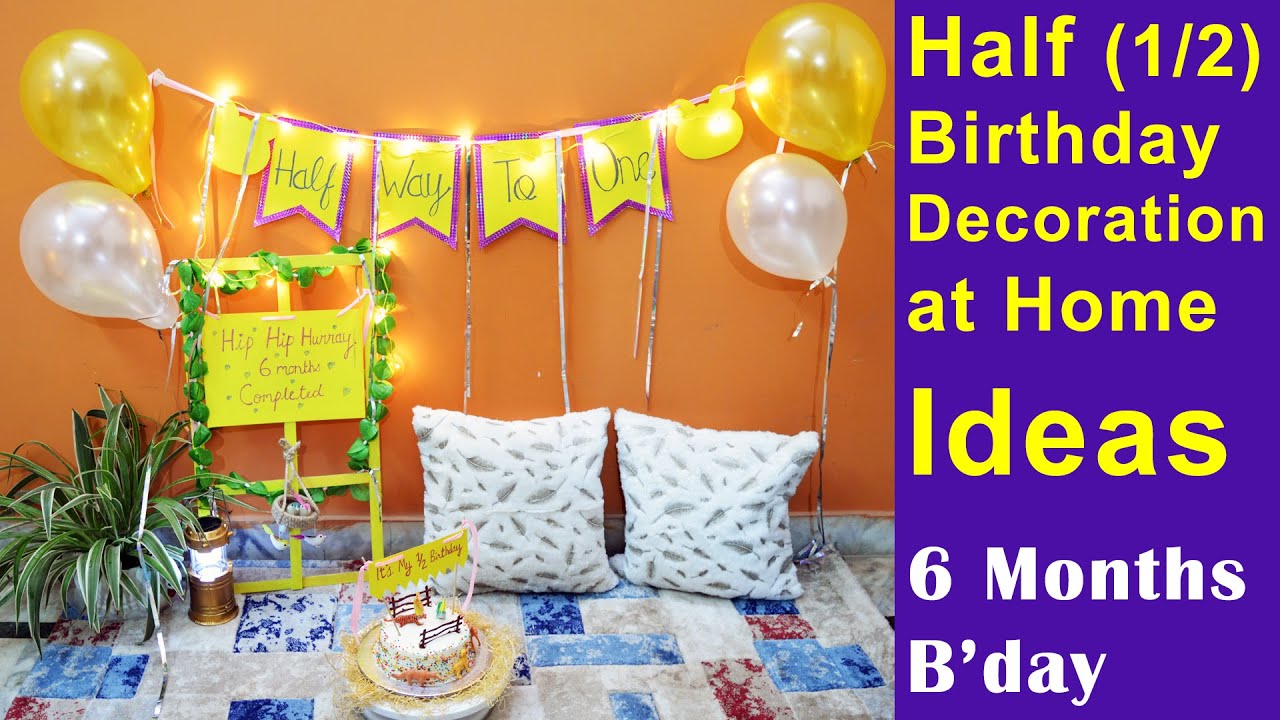The advertisement image for half birthday decoration ideas features a vibrant and festive scene set against an orange wall. A bold yellow banner with the words "HALFWAY TO 1" is strung across the wall, flanked by clusters of yellow and white balloons. Beneath the banner, a charming yellow frame adorned with viney green plants showcases a sign that reads, "HIP HIP HOORAY 6 MONTHS COMPLETED." The decor also includes fairy lights, adding a magical touch to the celebration.

On the floor, a multicolored rug featuring blues, grays, and reds adds a cozy atmosphere. Two white throw pillows rest nearby, next to a white cake decorated with small dinosaur figurines and a yellow topper that reads, "IT'S MY HALF BIRTHDAY" in red ink. Additional details include a pot plant on the left and a little basket next to the "HIP HIP HOORAY" stand.

To the right of the image, a purple section with yellow and white text reads: “HALF 1/2 BIRTHDAY DECORATIONS AT HOME IDEAS, SIX MONTHS BIRTHDAY.” This detailed setting provides a playful and creative inspiration for celebrating a six-month milestone at home.